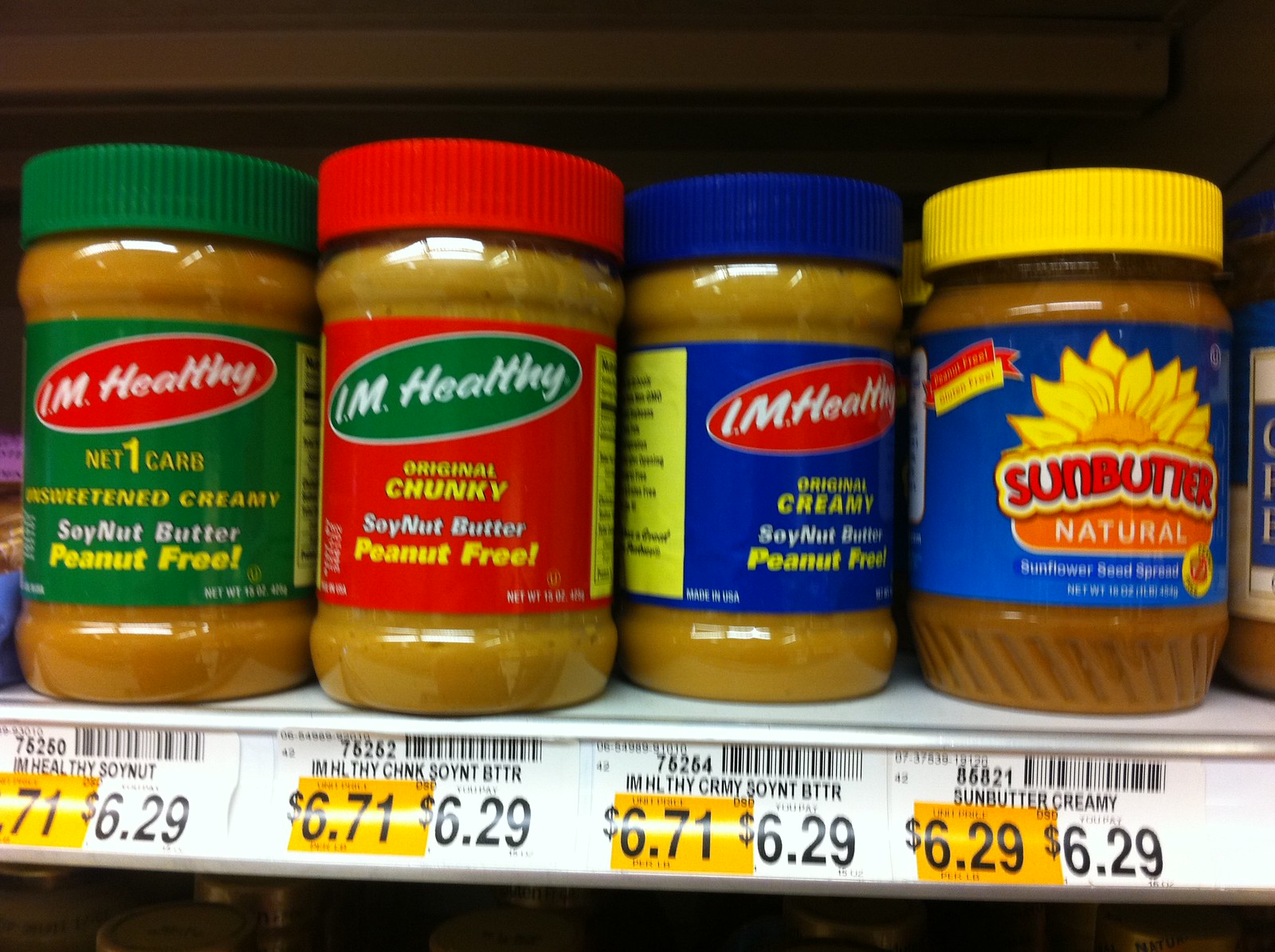This color photo captures a shelf in a grocery store, prominently featuring a lineup of four jars of nut butter displayed in a row. The shelf itself is white, accentuated by a series of black and white price tags at the bottom, with bright yellow highlighting behind the pricing, drawing immediate attention. Each translucent jar reveals contents of varying shades of brown, from a light caramel brown to a medium dark brown, offering a spectrum of nut butters.

On the far left, the first jar, with a green plastic lid and matching label, is identified as "Unsweetened Creamy Soy Nut Butter" and marked as peanut-free. The price tag below indicates a price of $6.29, possibly on sale. This is followed by a jar with a red top and label, labeled "Original Chunky Soy Nut Butter," also peanut-free, priced similarly at $6.29.

Next in line is a jar with a blue top and label, which reads "Original Soy Nut Butter," continuing the peanut-free trend and priced at $6.29. Finally, the jar on the far right stands out with a yellow cap and blue label, marked "Sun Butter Natural" with an illustration of a sunflower, identified as a good spread and also priced at $6.29.

The labels on the jars coordinate with their lid colors, enhancing visual appeal, while the clearly marked price tags below ensure easy identification for shoppers.